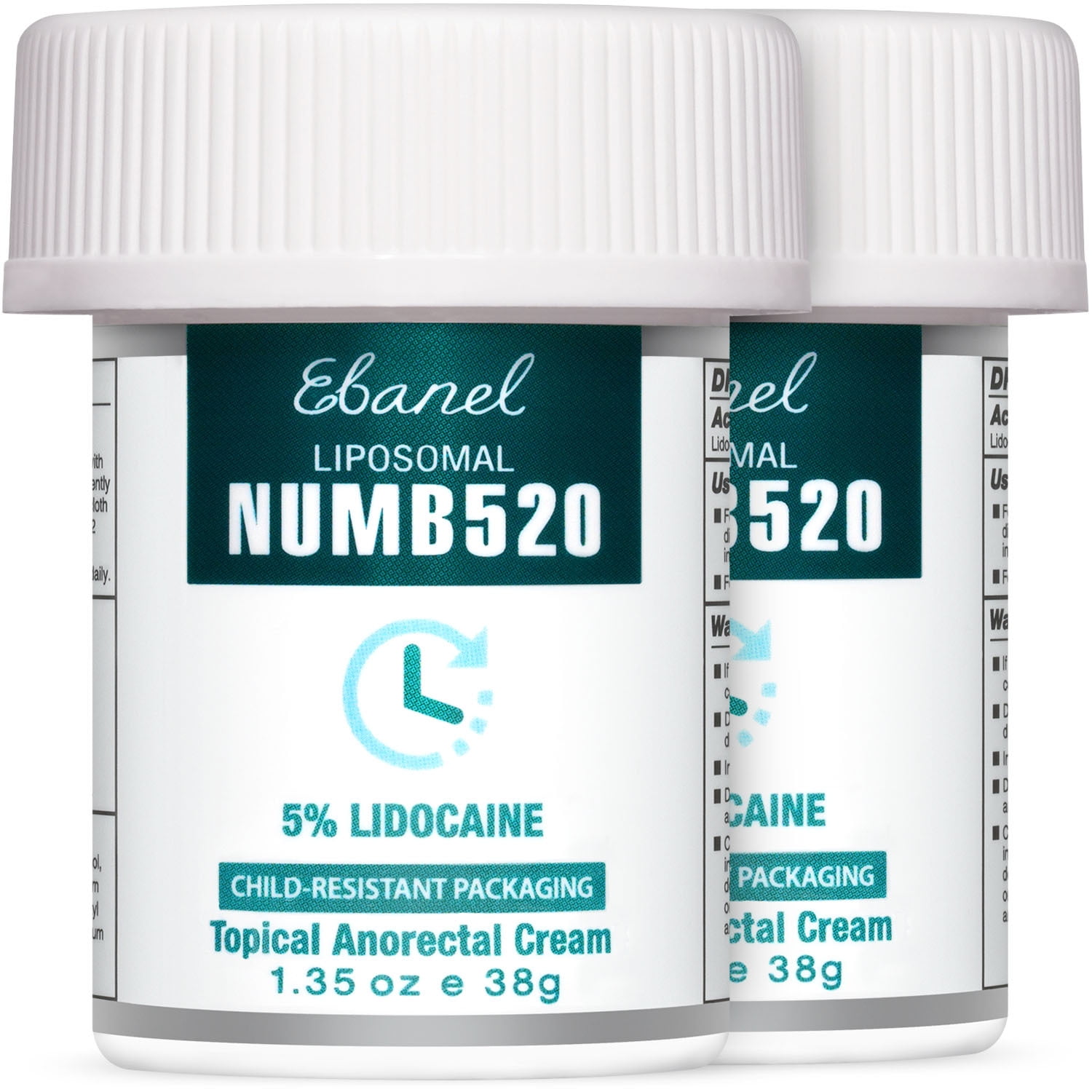This image depicts two small bottles of a topical anorectal cream. The bottles have wide, white, child-resistant safety caps and measure approximately an inch tall, each containing 1.35 ounces (38 grams) of the product. The labels are predominantly white with text and design elements in varying shades of blue or teal. At the top of each label, there is a green emerald square displaying the brand name "Ebenel Liposomal NUMB520." Below the brand name, there is an image resembling a clock, suggesting a time-release mechanism of the cream. Directly beneath the clock image, the labels indicate that the cream contains 5% lidocaine. Further down, it is clearly stated that this is a topical anorectal cream designed for specific medical needs.